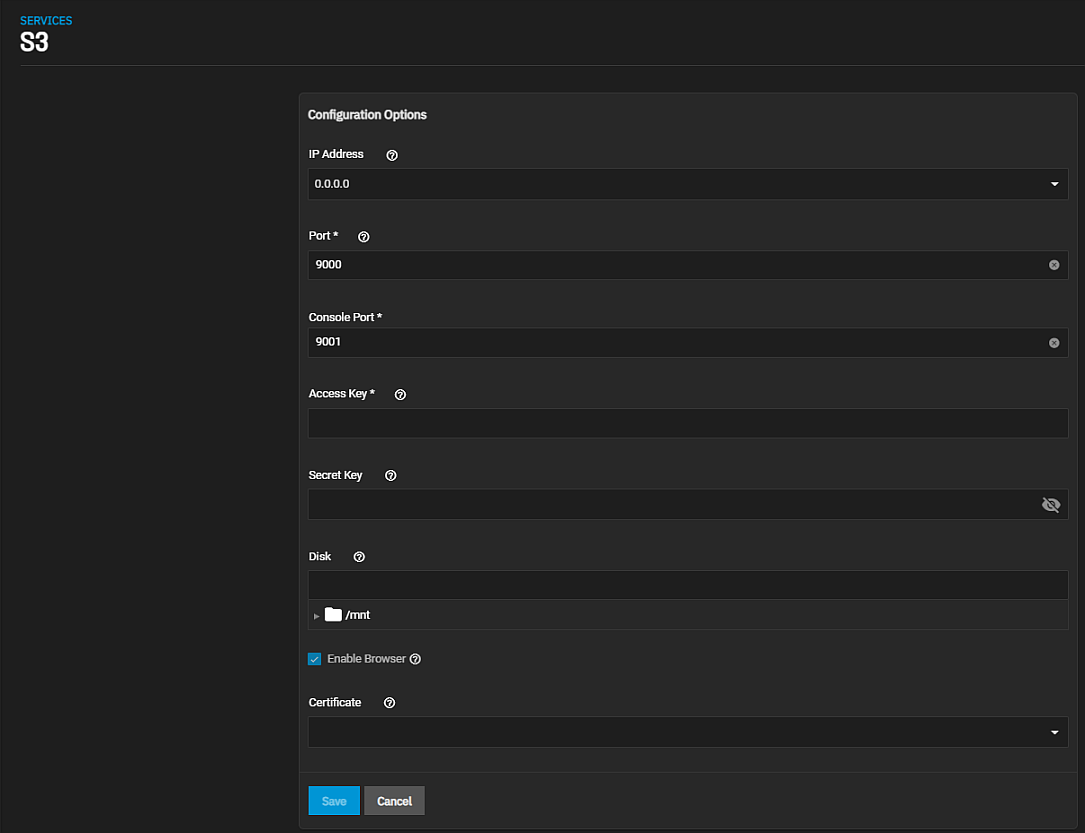In this image, we are looking at a screenshot with a solid black background. In the upper left corner, there is bold white text that reads, "services S3, S3." On the right side of the image, there are several gray boxes bordered with black at the top and the left side, containing white text.

The top section reads "Configuration Options". It includes fields such as "IP Address" with a black pull-down menu, "Port" with the value "9000", and "Console Port" with the value "9001". Below this, there are fields labeled "Access Key" and "Secret Key", both of which are blank. Adjacent to these fields, there is a small icon resembling a disk with a question mark.

Further down, there is a larger blank space within the box, followed by an icon of a file path designated as "/MNT". Lower down, a blue checkbox is ticked next to the text "Enable Browser". This is followed by a section labeled "Certificate."